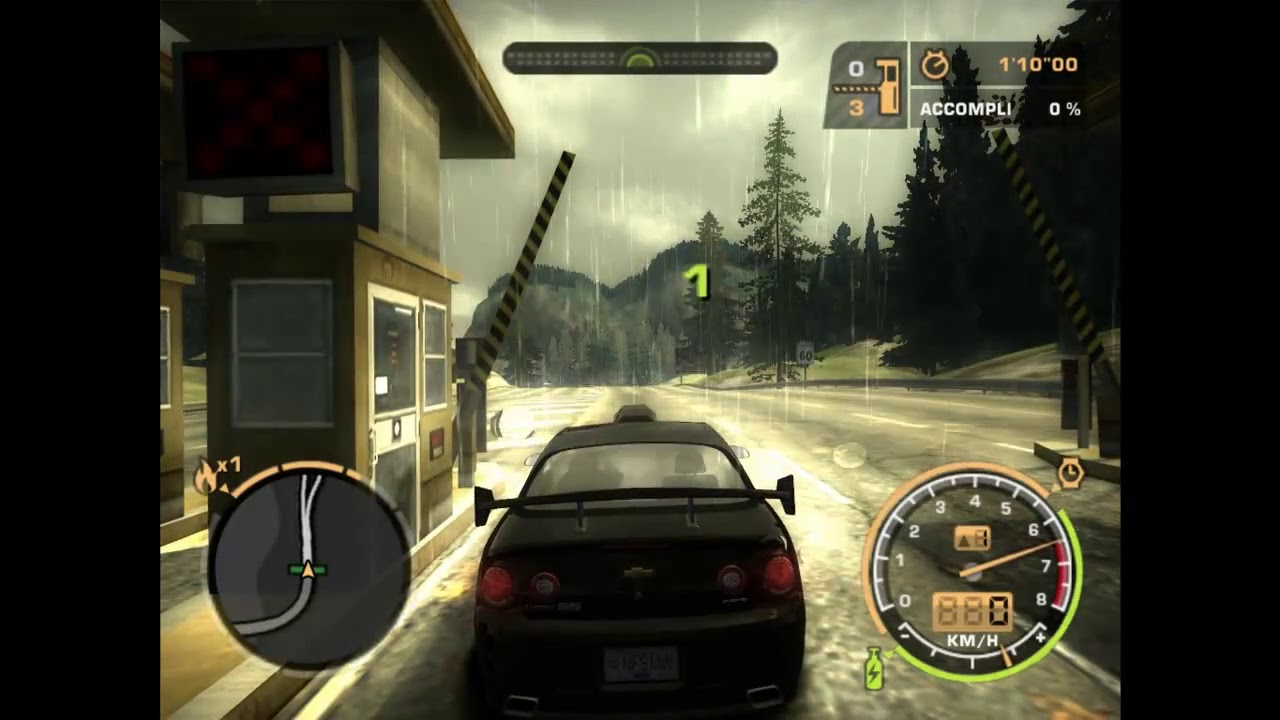The screenshot depicts a detailed scene from a video game that gives off strong Need for Speed or Grand Theft Auto vibes. The player's perspective is situated behind a meticulously rendered black Chevy Cobalt, complete with a license plate and a prominent spoiler. The car is approaching a toll booth with raised gates, poised to enter. One can discern a security guard's booth beside the entrance. The sky overhead is gray and gloomy, with rain adding to the dreary atmosphere. Lush green mountains and trees stretch across the background and to the right side of the image.

On the game's interface, several elements provide vital information: a circular GPS map is visible on the lower left, displaying the current road. To the lower right, a speedometer indicates the car's speed, while the upper right corner shows checkpoint details, including "0 out of 3" checkpoints completed, a timer reading "1:10", and 0% progress. In the middle of the screen, a green number "1" hints at a countdown or starting position. This level of detail suggests a complex driving experience, possibly including racing and open-world exploration elements.